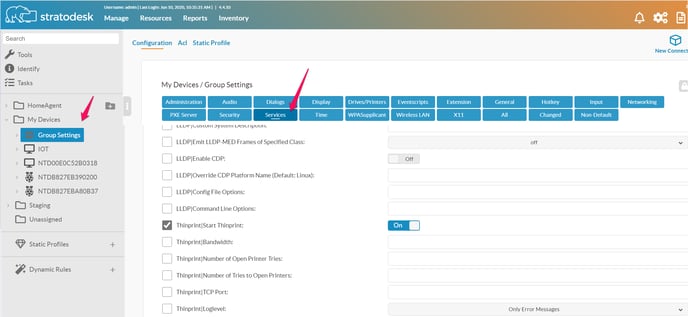A screenshot of the StratoDesk website is displayed, showcasing a vibrant and detailed user interface. At the top, a gradient border transitions from blue to green to brown to reddish-brown, contributing to the colorful theme of the site. Central to the interface is the StratoDesk logo featuring a polar bear at a computer.

The site’s navigation is robust, with links to "Home", "Agent", "My Devices", "Tasks", "Tools", and "Identity", all situated on the left side. Also on the left, a menu prominently displays options such as "Configuration", "Add", "Static Profile", and "Group Settings", the latter highlighted in blue. There’s also extensive detail here, with numerous sub-options listed and various computer-related items.

In the body of the webpage, the content is more minimalistic. It contains several boxes, one of which is marked "On" in blue with white text. Another element includes a checkbox, filled with a white tick inside a gray square.

Icons in a brownish hue appear on the right side, yet the right section’s text is sparse. The interface also features a search bar for ease of navigation. Overall, the screenshot highlights a sophisticated and colorful design with a focus on functionality and detailed configuration options on the left, with a simpler, less populated right-hand side.